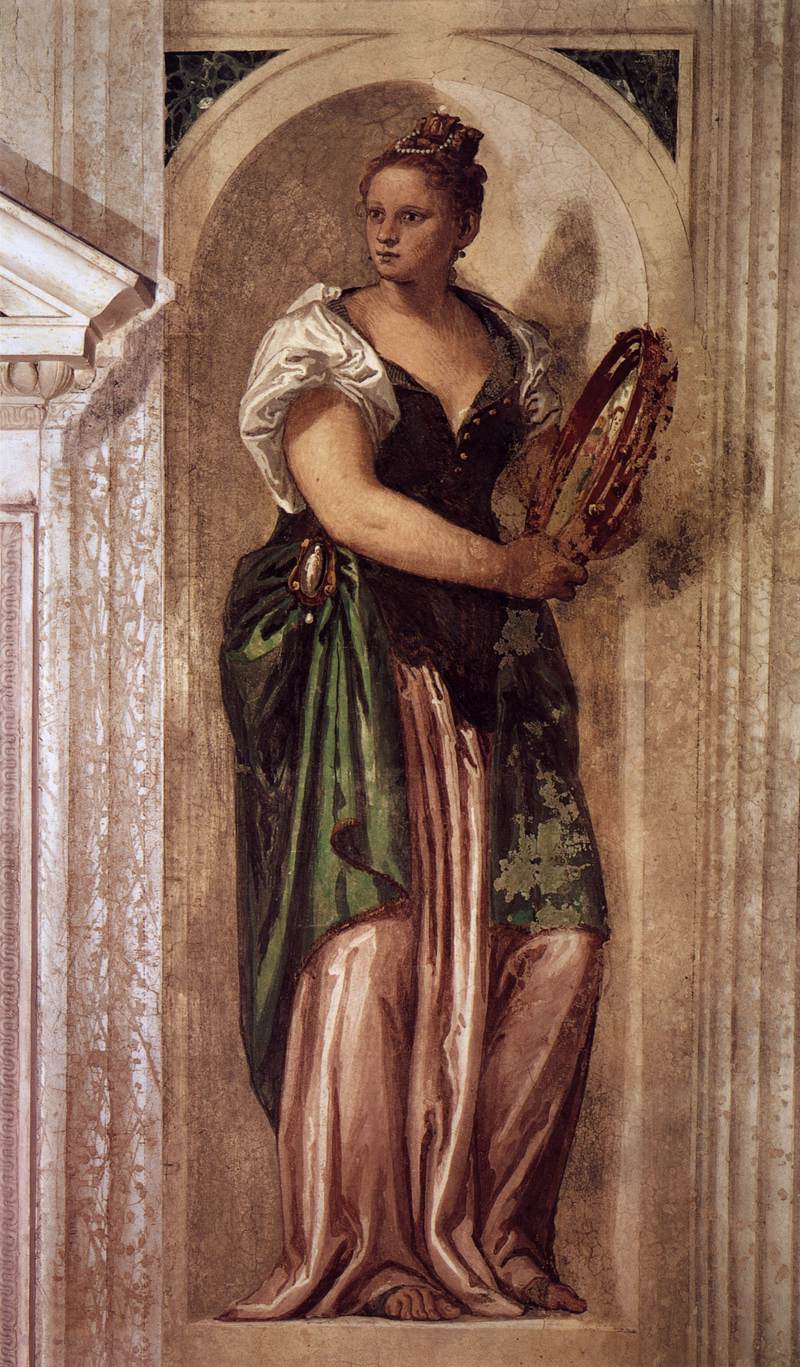This vertically rectangular image captures a detailed photograph of a statue inside a building, likely made of marble or a similar stone. The central figure is a woman standing on a small platform within a stone niche, which is arched at the top and flanked by brownish-beige stonework with a triangular structure visible on the left. Her attire consists of a green dress with buttons on the chest area, and it flows down to cover her bare feet, with the lower part being a brown color. The sleeves of her dress are ruffled and ivory-colored, and her upper chest is bare. She has puffy sleeves with bare arms and her hair, which appears to be light brown or reddish-brown, is styled in curls piled on top of her head, adorned with a necklace. The woman’s gaze is directed towards the left side of the image, though her body faces the right. She holds a circular brown object, which could be a tambourine or the top of a tennis racket, with both hands. The statue is set against a background that appears brownish-beige, giving the image a vintage feel. No additional objects, borders, words, or numbers are present, ensuring the focus remains solely on the intricately detailed statue.